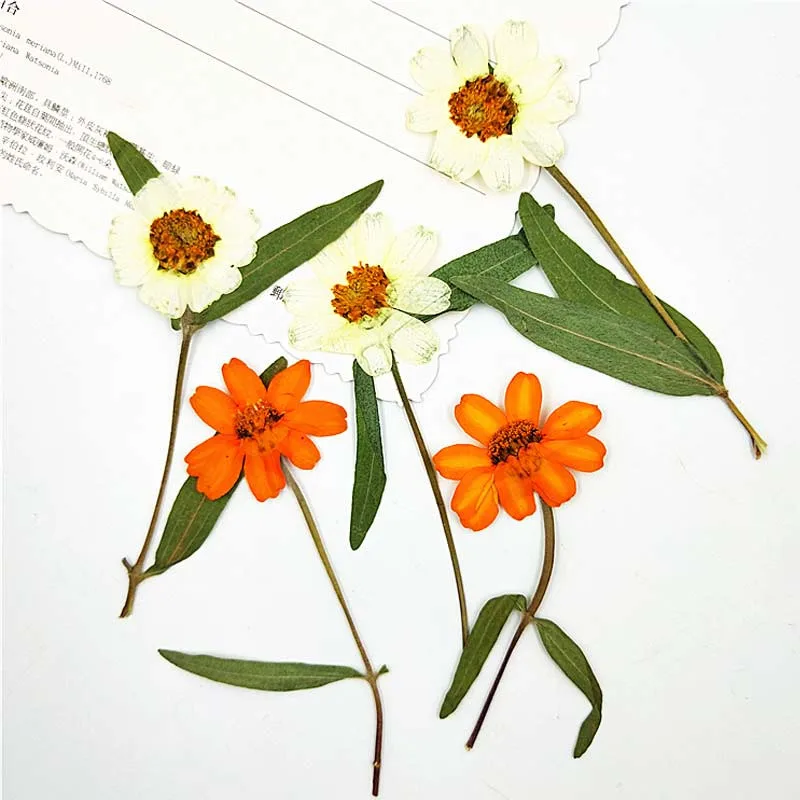The photograph showcases a delicate arrangement of five dried, pressed flowers against a stark white background, with a partial view of a document or postcard featuring Chinese lettering in the top left corner. Three of the flowers, positioned centrally and overlapping the postcard, have white petals with vibrant orange stamens at their centers. These blooms resemble daisies and are flanked by long, skinny green leaves. Below these white flowers lie two additional blooms, characterized by their oblong reddish-orange petals and similarly orange stamens. Each of the flowers is intricately preserved, with the white flowers displaying approximately ten petals each. The arrangement of the pressed flowers and the partially visible document with Chinese text creates a harmonious and sentimental composition, suggesting the flowers were carefully dried and kept as a cherished memento.